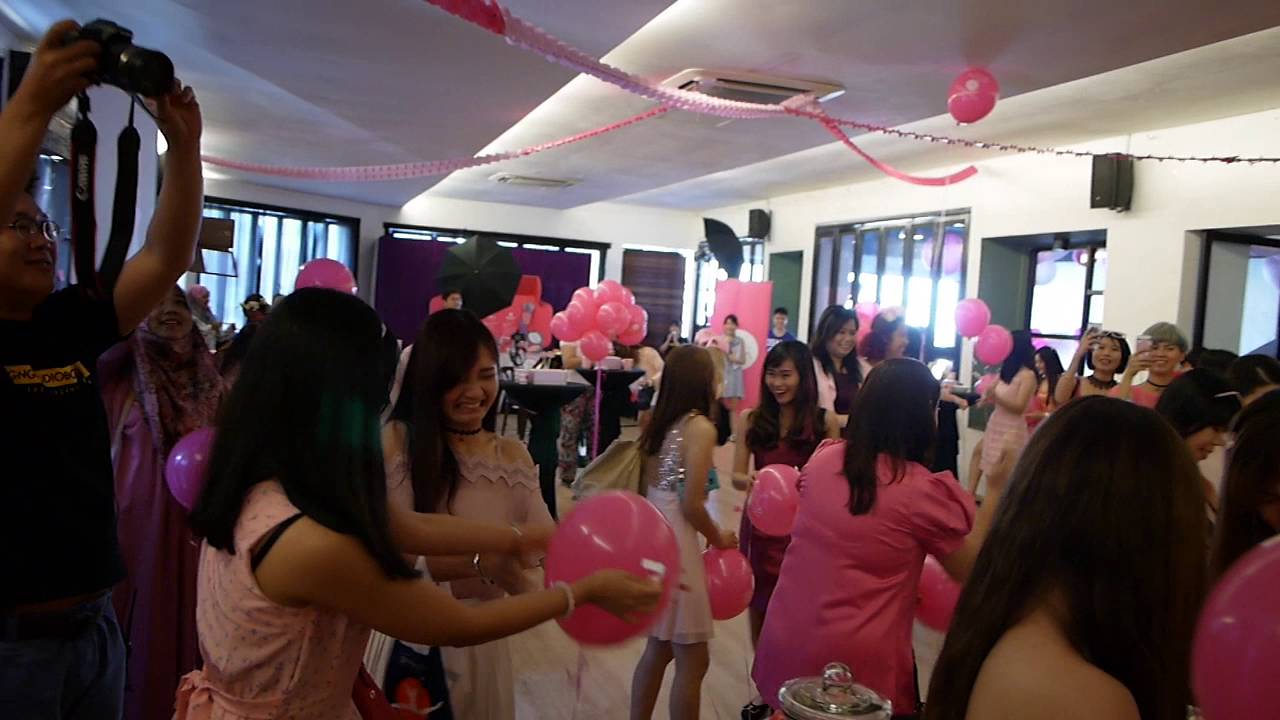In a lively party filled with joy and laughter, a room adorned with an abundance of pink decorations comes to life. The partygoers, predominantly women with long, straight dark-to-black hair and Asian features, are dressed in a variety of pink shades, ranging from ballet pink to hot pink, creating a vibrant and cohesive atmosphere. The event, possibly a Hindu celebration or gender reveal, takes place in a spacious area with floor-to-ceiling windows that allow natural light to flood the room, highlighting the light brown hardwood floors.

At the center of the room, a striking bouquet of bright pink balloons captures the attention, while numerous other pink and plum-colored balloons add to the festive ambiance. Guests are seen gleefully playing with the balloons, attempting to pop them and capturing these fun moments on their phones. A man in a black t-shirt and dark blue pants, standing towards the left, is prominently featured holding a Canon camera above his head, documenting the various activities.

In the background, a well-lit photography setup with studio lighting and a big purple curtain, along with an umbrella for camera flashes, is arranged to take professional photographs of the guests. Alongside, what seems to be a DJ adds to the party's energetic vibe. The walls and ceiling are painted white, serving as a neutral backdrop that enhances the festive pink theme of the celebration. The guests, including a lady in a Muslim head covering and several women with mid-length brown hair, all exude happiness, thoroughly enjoying the cheerful and colorful gathering.